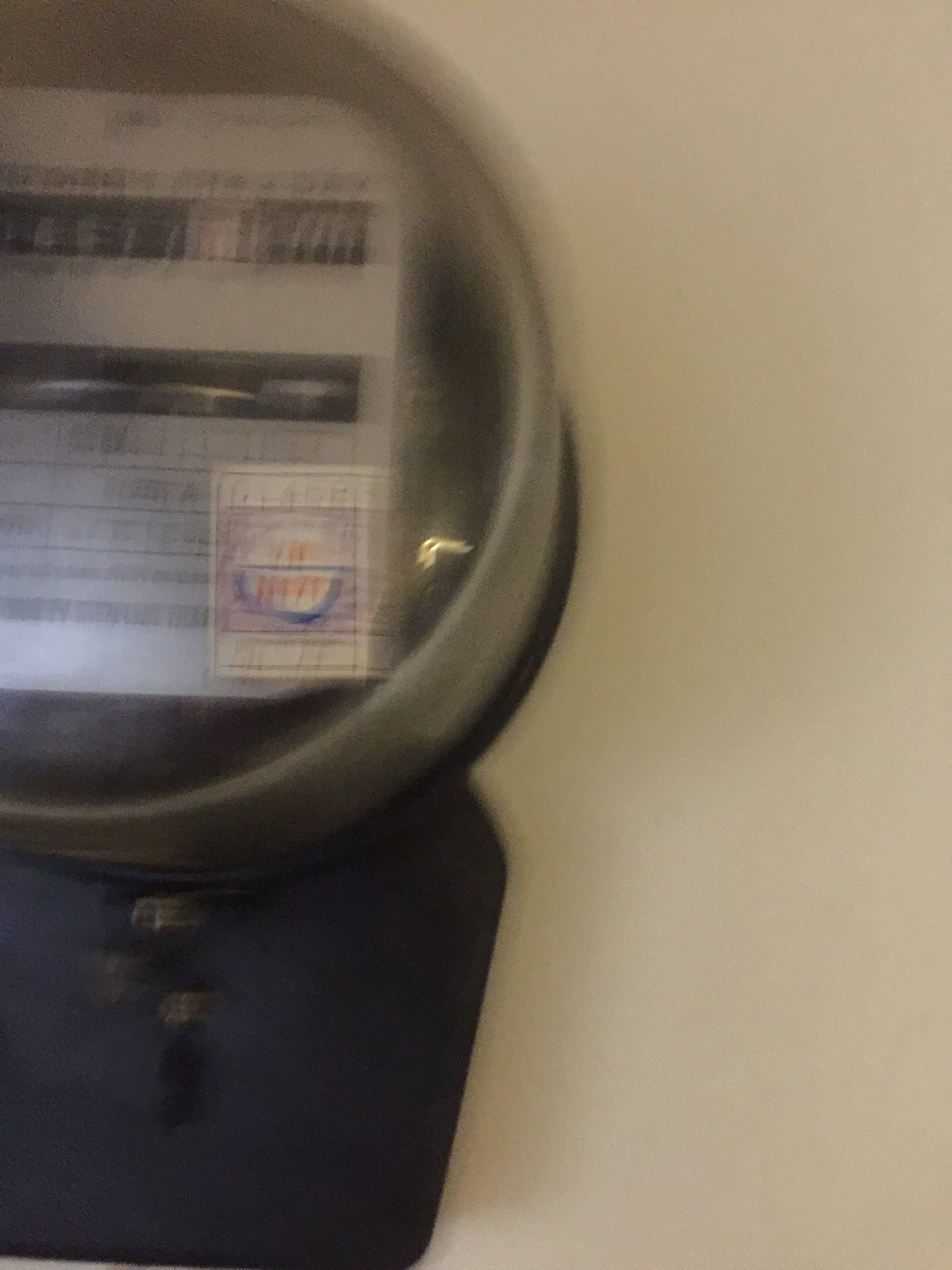This photograph captures a slightly blurry image of a circular electric meter, likely positioned inside a unit such as a garage, laundry room, or closet. The meter, which could have been photographed with a DSLR or smartphone camera, has a clear plastic cover allowing the readings to be visible. The exterior of the meter features a black base and some elements in light gray. Below the meter, there is a dark blue rectangular piece, possibly a cloth. Inside the meter’s plastic enclosure, a gray piece of paper with blurred handwriting and some stickers is visible. One of the stickers is a small white square with blue and orange details, while another is violet with dark blue and red text. The image lacks human presence and shows a light gray background, which could be the surface or wall of the area where the meter is installed.